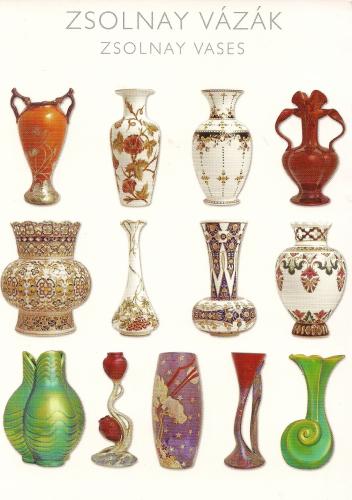This image features an arrangement of 13 exquisitely designed vases, displayed on an eggshell white background. The setting looks like a product poster. The name "ZSOLNAY VAZÁK" is prominently featured in gray text at the top center of the image, with "ZSOLNAY vases" written in smaller text below.

The vases are organized into three rows: four vases in the top and middle rows, and five in the bottom row. The top two rows showcase more traditional and classical designs, exuding a regal and sophisticated aesthetic. These vases vary from large urn shapes to more slender, narrow forms. Some feature elegant handles, while others do not.

The bottom row presents eclectic and abstract designs, including a particularly unique rose-shaped vase, second from the left. The vases are diverse in their appearance, boasting vibrant colors such as green, red, gold, and white, and often adorned with intricate floral motifs. Some have iridescent glass treatments, like one which transitions from green to yellow, and another, which resembles a snail shell with a green iridescent finish that opens into a fluted top.

Overall, the vases reflect a rich array of embellishments and patterns, some rendered in etched gold, making them look like precious items that one might find in a museum or for sale in an exclusive gallery.